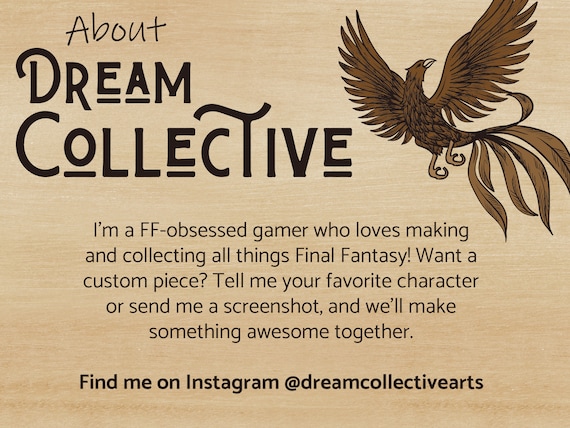This digital advertisement for Dream Collective features a striking bird creature, possibly a phoenix, prominently displayed in the top right corner. The bird is depicted in mid-flight, showcasing its outstretched wings and long, elegant feathers, both in its wings and tail. The creature is rendered in a rich, darker brown color. Against a light wood or tan-colored background, which gives the appearance of text burned into the surface, the poster includes an extensive promotional message. It reads: "About Dream Collective. I'm a Final Fantasy (FF) obsessed gamer who loves making and collecting all things Final Fantasy. Want a custom piece? Tell me your favorite character or send me a screenshot and we'll make something awesome together. Find me on Instagram at Dream Collective Arts." This meticulously detailed piece not only serves to highlight the artist's skill in creating fantasy-themed art but also promotes their Instagram account and custom artwork services tailored for fans of the Final Fantasy series.